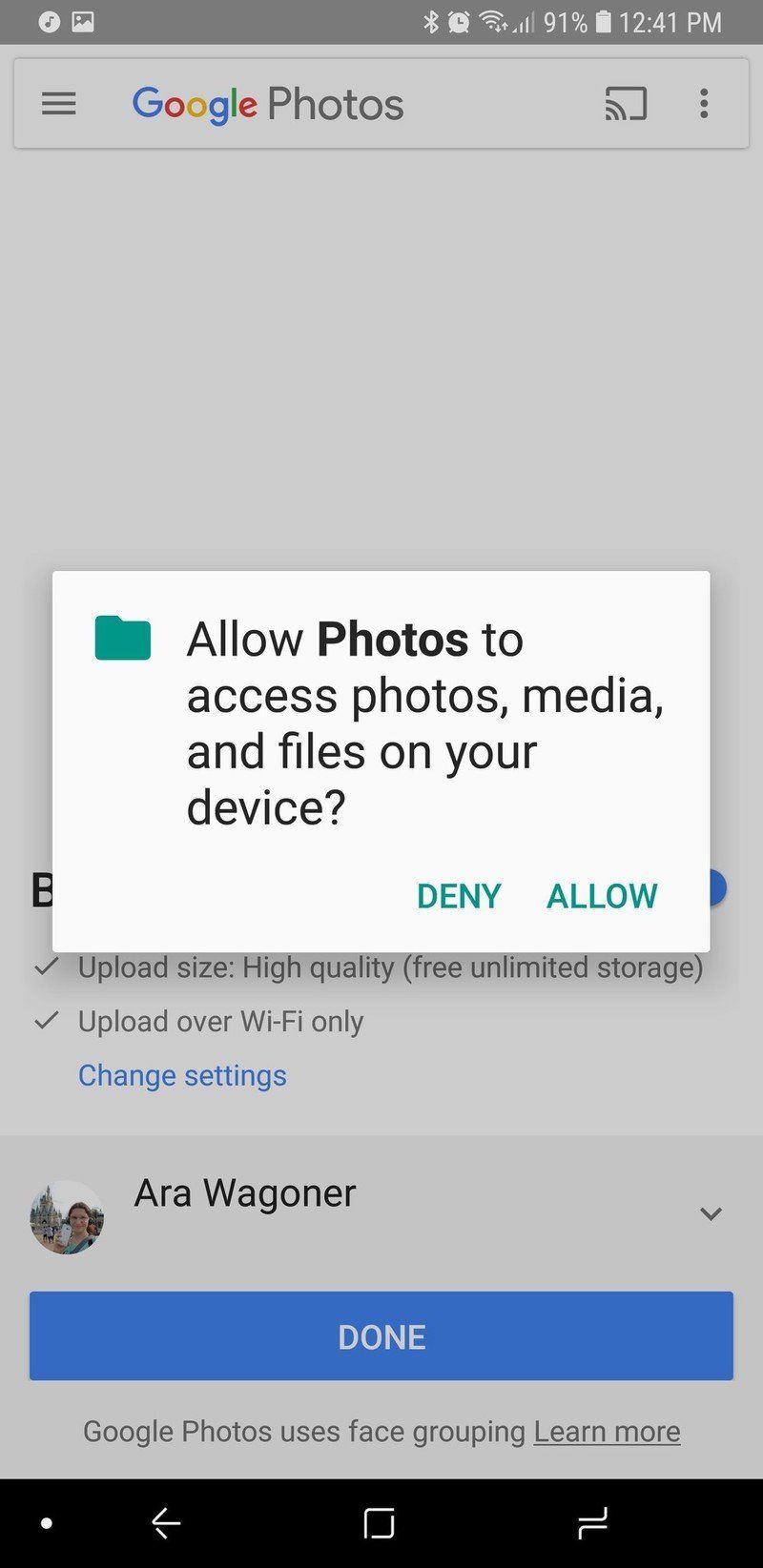This is a detailed screenshot from the Google Photos app on a mobile device, belonging to a user named Ara Wagoner. The app interface displays a pop-up message prompting the user to "Allow Photos to access photos, media, and files on your device." This message gives the user the option to either "Deny" or "Allow" access, with the respective buttons highlighted in green. At the bottom of the screen, there is a "Done" button. Beneath this, the device's navigation bar is visible, featuring a back arrow button, a home button, and an unidentified third icon. The backdrop of the screenshot is the typical Google Photos interface.